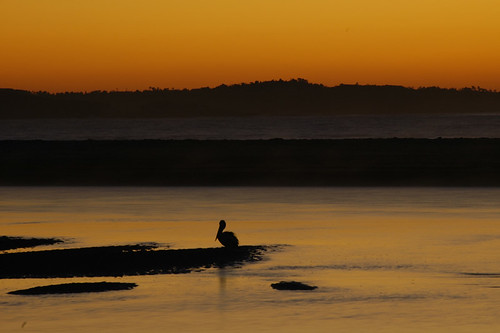In this captivating outdoor nature scene, the beauty of a sunset or sunrise is magnificently captured. The sky radiates a dark orange hue, painting a serene backdrop. In the foreground, tranquil water mirrors the sky's glow with a subtle orange tint overlaying its gray surface. Light glimmers gently on the water, creating a nearly magical ambiance.

On the left side, a small piece of land juts into the water, providing a perch for a solitary pelican. The pelican, facing left, rests its long beak against its chest, showcasing its rounded body while its legs remain hidden from view. The water below reflects the pelican's silhouette, adding depth to the scene.

In the background, the silhouetted outline of the opposite shore forms a dark contrast against the illuminated sky. Trees line this distant shore, their shapes barely discernible beneath the vibrant orange sky above, completing this picturesque tableau of nature's splendor.